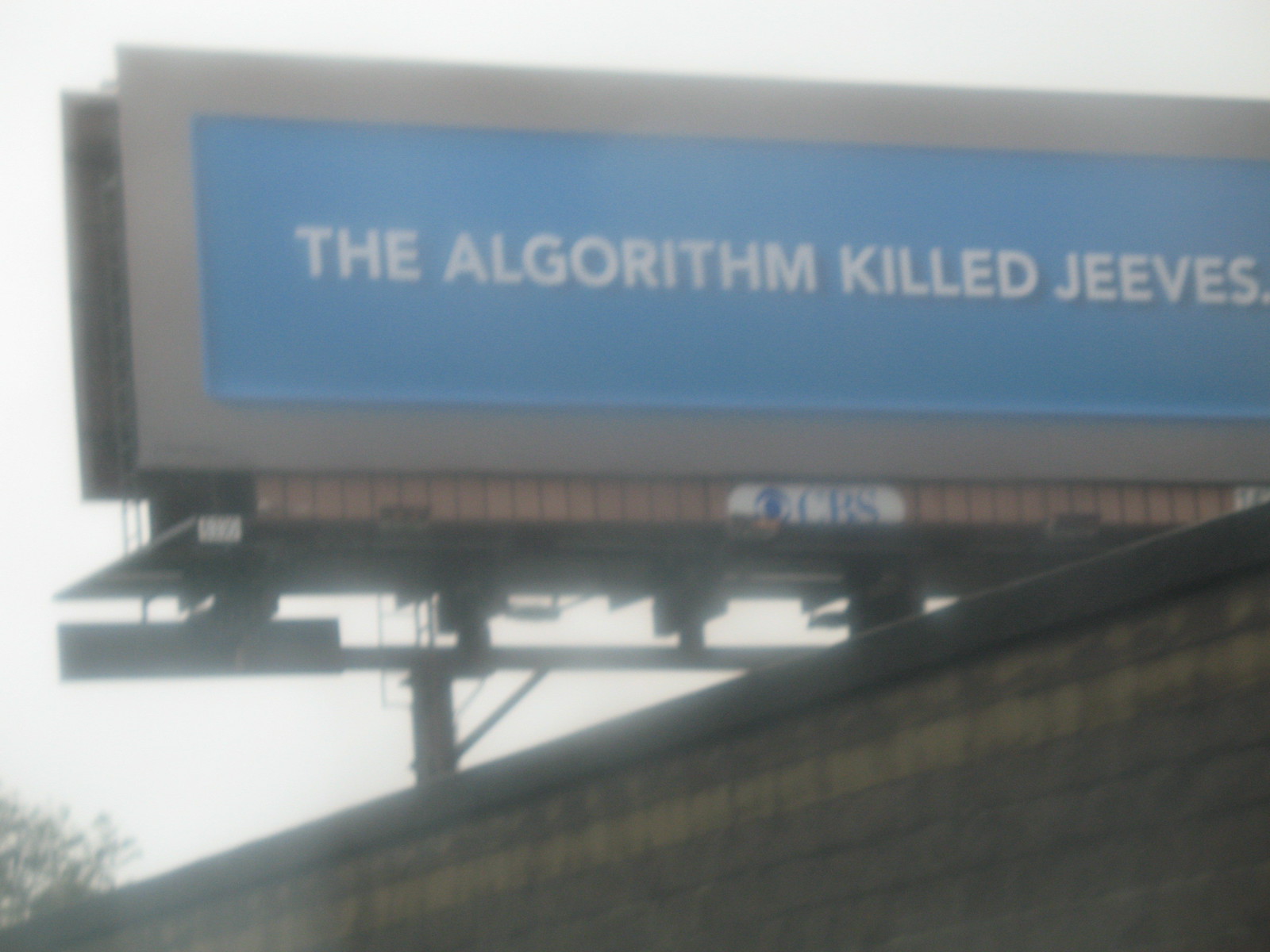The image depicts a large billboard mounted on the side of a gray building with a faint yellow stripe at the top. The billboard has a grayish-silver border framing a medium blue background, similar to a North Carolina blue. In bold, all-capital white letters, it reads, "THE ALGORITHM KILLED JEEVES." This phrase references the old Ask Jeeves search engine. Below the billboard, there is a small sign with the CBS logo, featuring white text on a blue background and the CBS eye emblem. The surroundings show a gray, overcast sky, a treetop peeking from the bottom left corner, and what appears to be a roadway or wall at the bottom of the photograph. Additionally, there is some wood paneling and wiring visible just beneath the billboard.